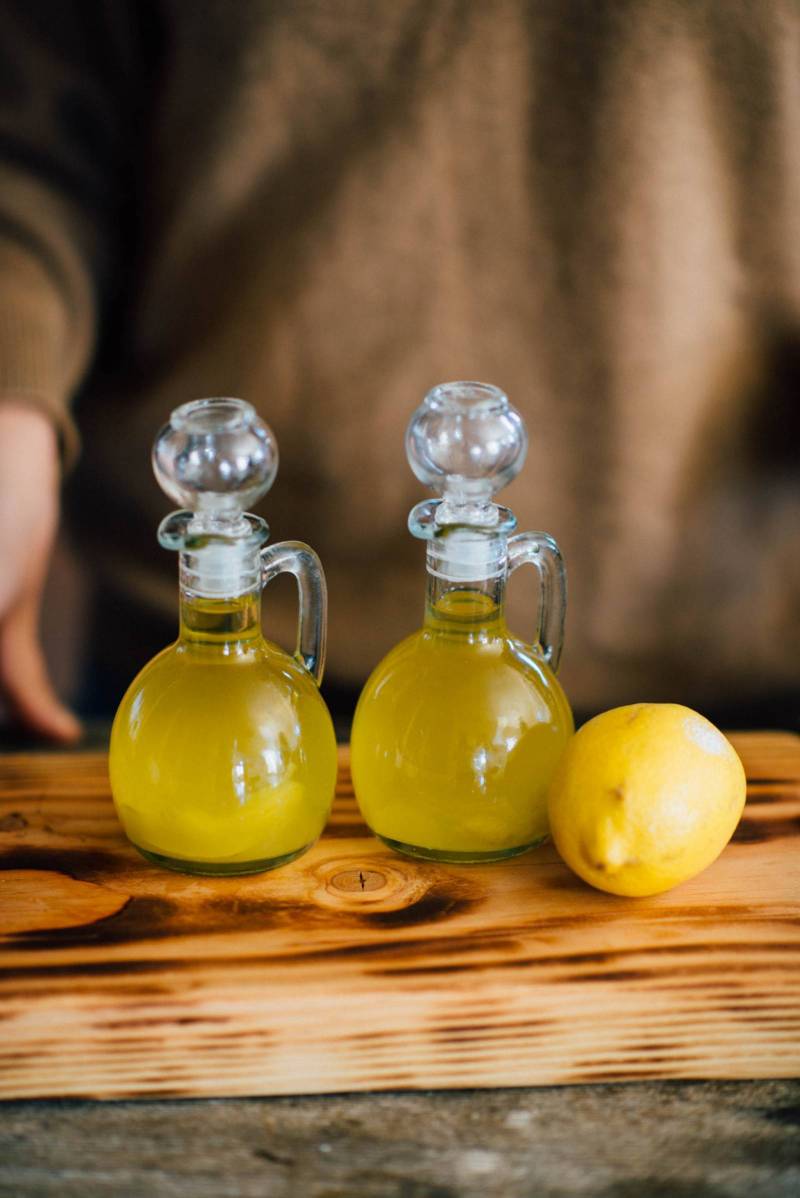This vertical photograph, reminiscent of a cookbook illustration, showcases two identical glass bottles filled with what appears to be a lemon-infused olive oil. Each bottle has a spherical glass stopper, a handle, and a slender neck that expands into a round, snow globe-like base with a flat bottom. Positioned to the right of these bottles is a fresh lemon. Both the bottles and the lemon are placed on a light wooden cutting board accented with dark wood details, which rests on a gray countertop. In the background, a person clad in a brown sweatshirt is partially visible, with their torso and a portion of their hand subtly framing the scene.